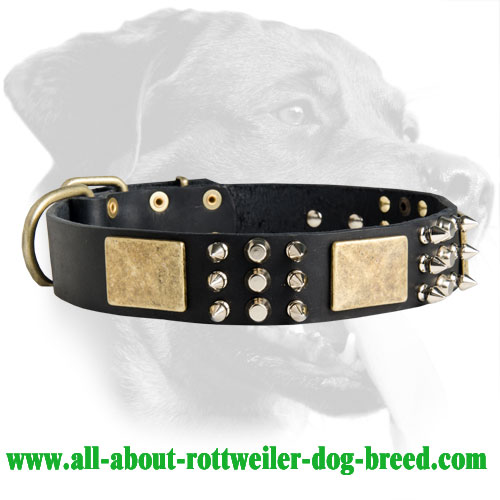The image features a faded, black-and-white photo of a Rottweiler in the background, giving it a ghostly appearance. Overlaid on this subdued dog image is a striking collar, which appears to either float in the air or rest flat with no visible surface. This ornate collar is likely made of black leather and is adorned with an array of decorative elements: it has three rows of three sparkling, gem-like studs resembling diamonds, flanked by two gold square accents. Additionally, the right side of the collar boasts intimidating, spike-like protrusions. This ensemble exudes an air of toughness and aggression. At the bottom of the image, the website "www.all-about-rottweiler-dog-breed.com" is displayed in green text, with hyphens separating each word. The overall layout combines a spooky dog image with an equally imposing collar, creating a bold and edgy advertisement.